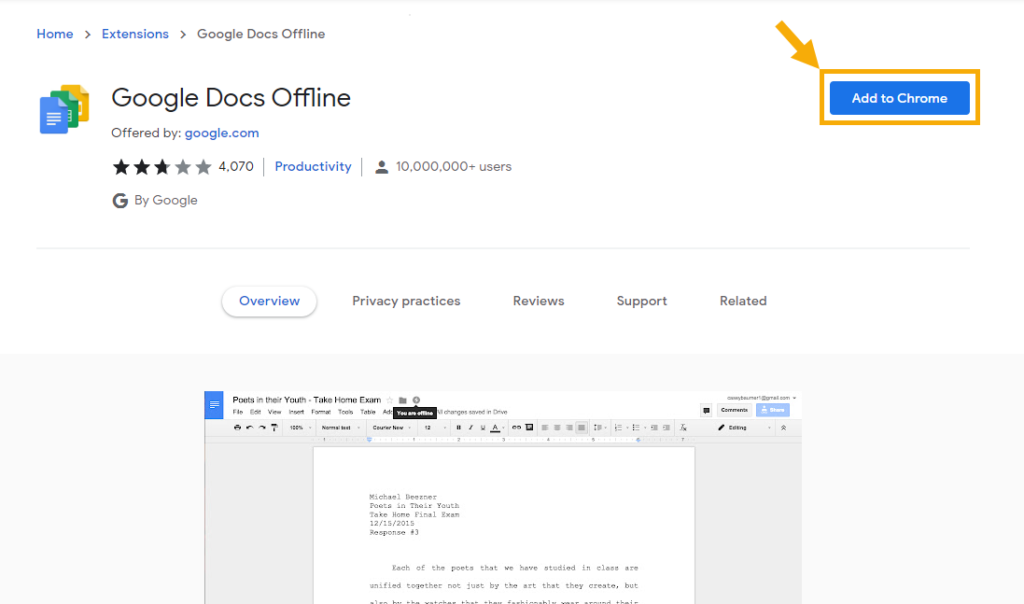The image displays a computer screen with a white background featuring a web page dedicated to Google Docs Offline on the Chrome Web Store. At the top left corner, "Home" is written in small blue letters, followed by a right caret, then "Extensions" also in blue, another right caret, and finally "Google Docs Offline" in gray letters. Below this, to the left, there is an icon consisting of three stacked rectangles in blue, green, and yellow, resembling sheets of paper.

Next to the icon, in larger black letters, it says "Google Docs Offline". On the same line to the right, there is a rectangular blue button with white letters that read "Add to Chrome". This button is highlighted by a gold-colored rectangle and an accompanying gold arrow pointing from the top left towards the button's top left corner.

Underneath the large "Google Docs Offline" text, in smaller letters, it states "Offered by google.com." Below this, there is a rating displayed with three out of five stars and "4070 ratings." It’s indicated in blue letters that the app is categorized under "Productivity" and has "10,000,000+ users." Further below, a large letter "G" is accompanied by the words "By Google". 

A thin gray line runs horizontally across the screen, below which there are four clickable options: "Overview" highlighted in a white oval button with blue letters, and "Privacy practices," "Reviews," "Support," and "Related," all in gray type.

Further down, a section of a Google Docs screen is visible, showcasing an editable document titled "Poets in Their Youth Take Home Exam." The top menu includes standard document editing options: "File", "Edit", "View", "Insert", "Format", and "Tools." A button indicating "You are offline" is also present. The sample document preview features the title "Michael Biesner Poets in Their Youth Take Home Final Exam 12-15-2015 Response Number Three," with the beginning of Michael Biesner's response: "Each of the poets that we have studied in class are unified together not just by the art that they create but..." before the text cuts off.